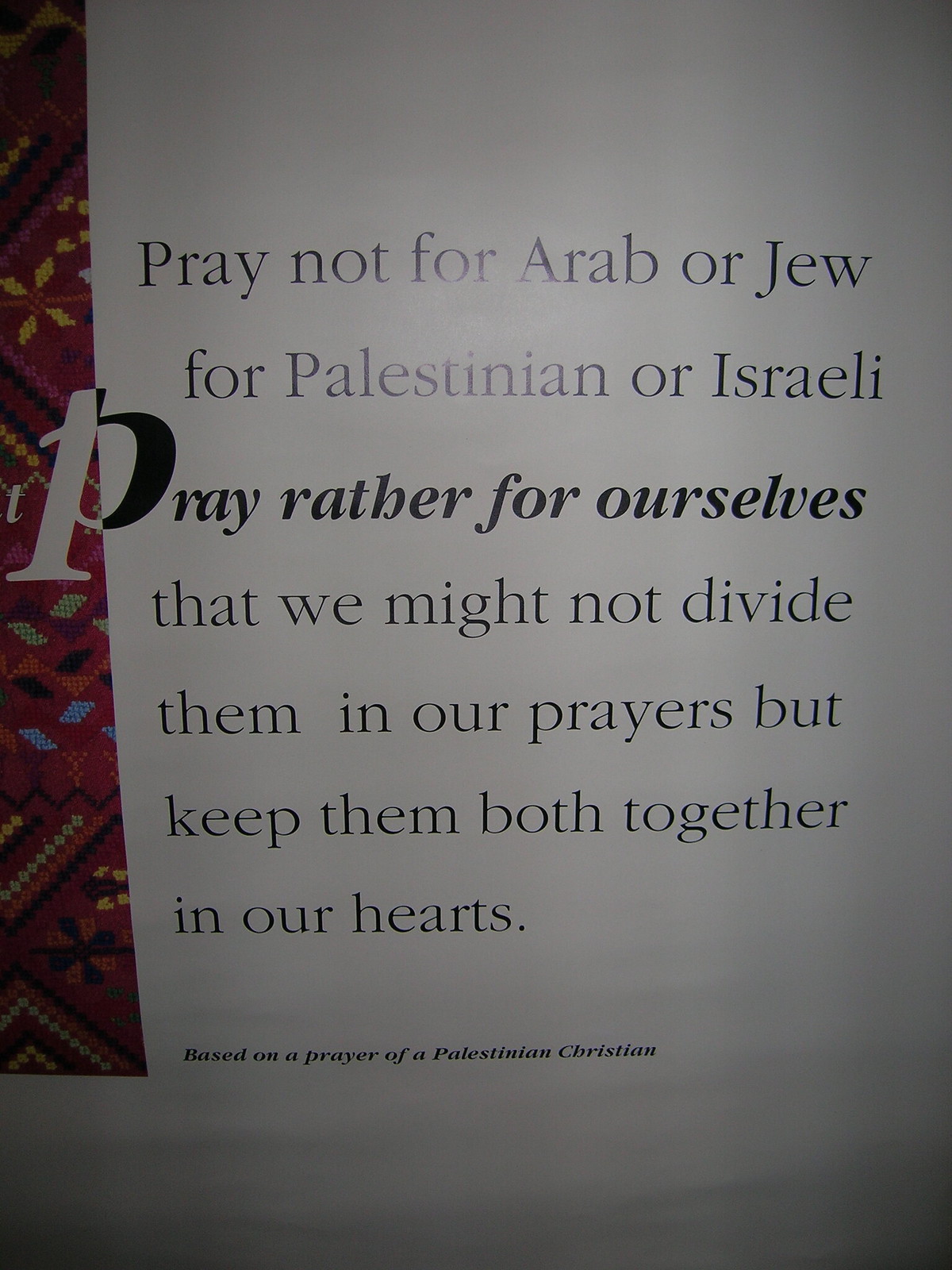The image depicts a white piece of paper or a page, featuring a meaningful message based on a prayer of a Palestinian Christian. The text, predominantly in black with certain parts italicized, reads: "Pray not for Arab or Jew, for Palestinian or Israeli, pray rather for ourselves that we might not divide them in our prayers, but keep them both together in our hearts." Notably, the phrase "pray rather for ourselves" is bolded for emphasis. On the left side, there is a flowery, quilt-like design with a red background and patterns composed of various colors including green, blue, yellow, and black. The overall appearance of the image is that of a thoughtful and artistic presentation, combining poignant words with intricate designs.